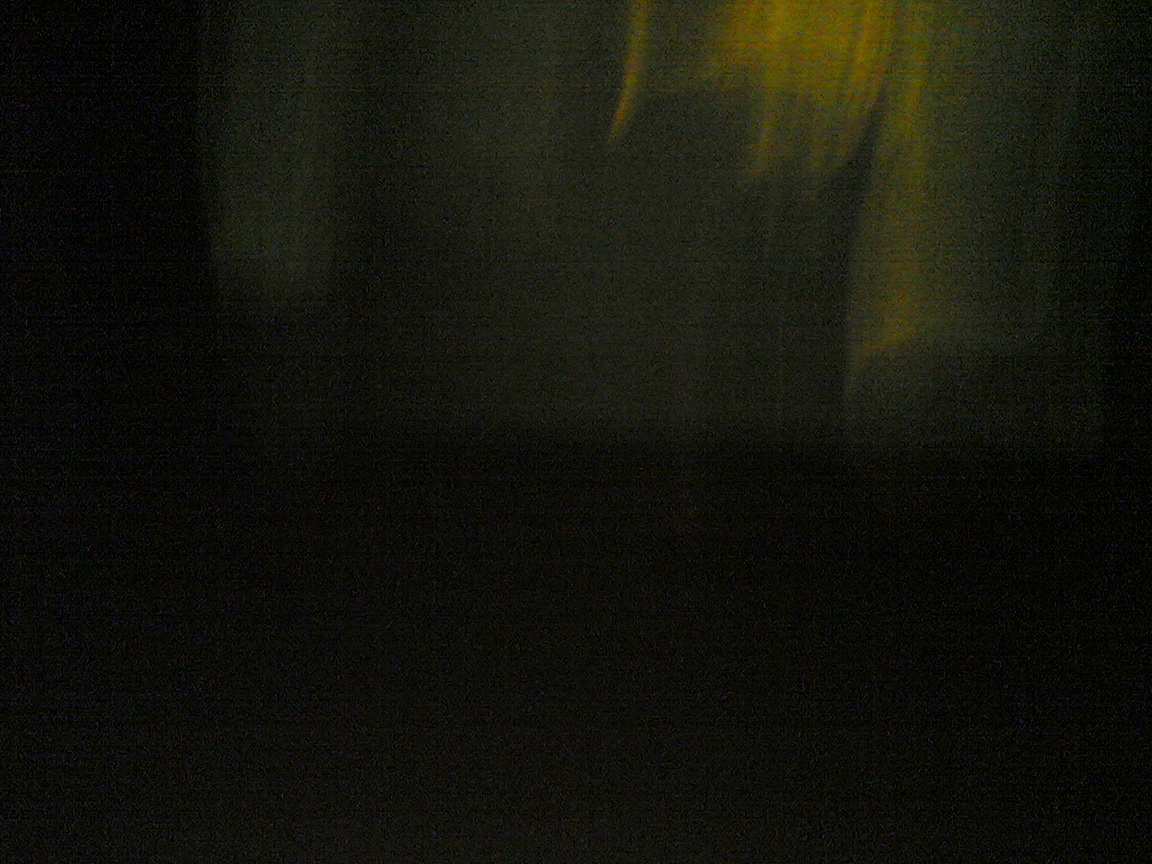A completely black square occupies the entirety of the frame. The image is devoid of any additional elements—there are no objects, text, or other colors present. The black box is perfectly square, with a uniform, uninterrupted blackness that lacks any detail or variation. The absence of features makes the image stark and minimalistic, focusing solely on the deep, rich black color that fills the square.